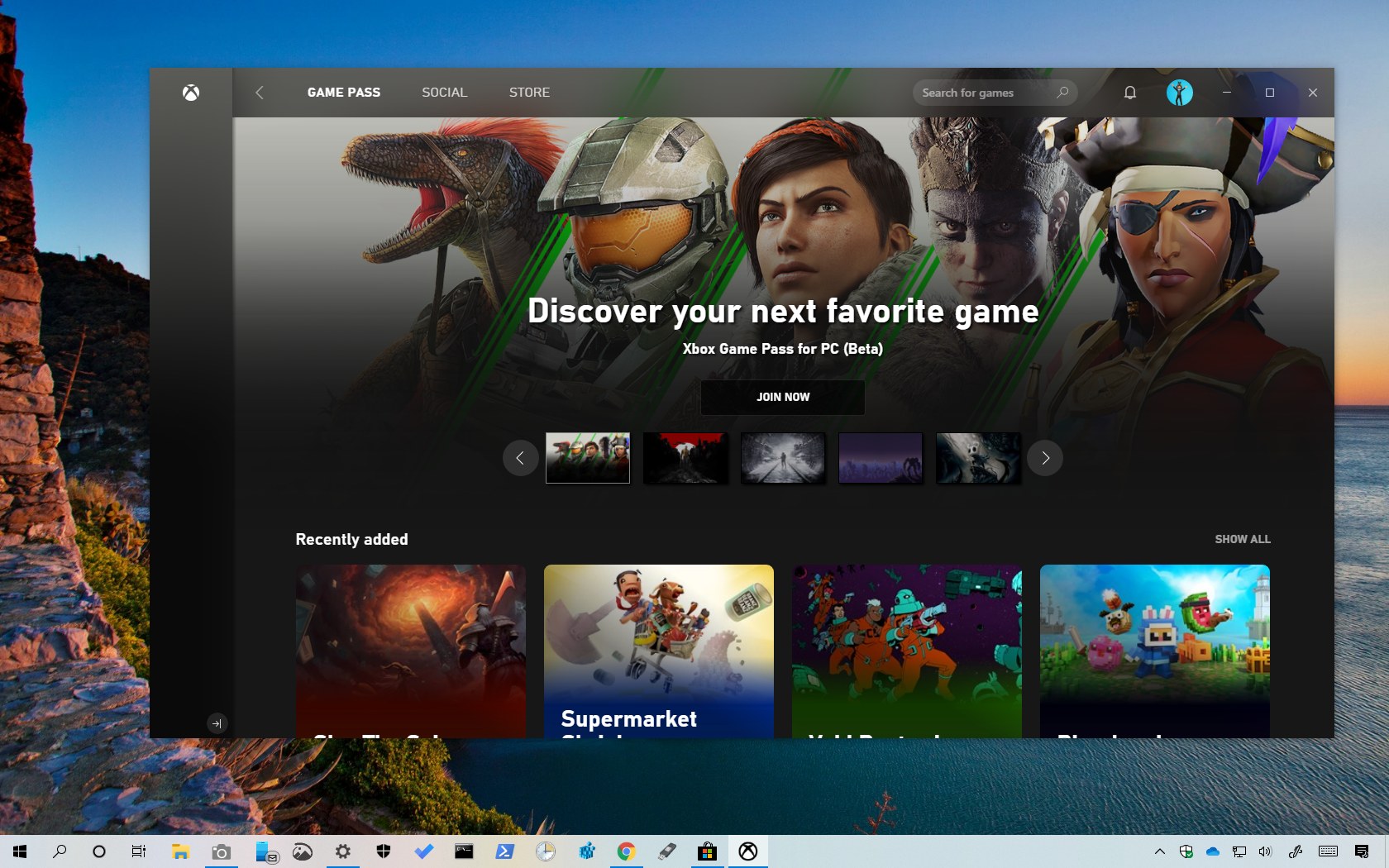The image is a screenshot of a Windows desktop. The taskbar at the bottom is a light blue color and shows various icons, including one with the Xbox logo that has been selected. The background is a serene nature or seascape wallpaper, depicting the ocean at sunset with a rocky shoreline and cliffs on the left. 

Occupying approximately 80% of the screen is the Xbox Game Pass window. This window has a dark background and features the header "Game Pass" at the top, along with tabs labeled "Social" and "Store." The "Game Pass" tab is currently highlighted. Below the header is a visually striking banner showcasing different video game characters, including a dinosaur, the Master Chief from Halo, a pirate, and two other unidentified characters. Accompanying the banner is the text: "Discover your next favorite game. Xbox Game Pass for PC Beta."